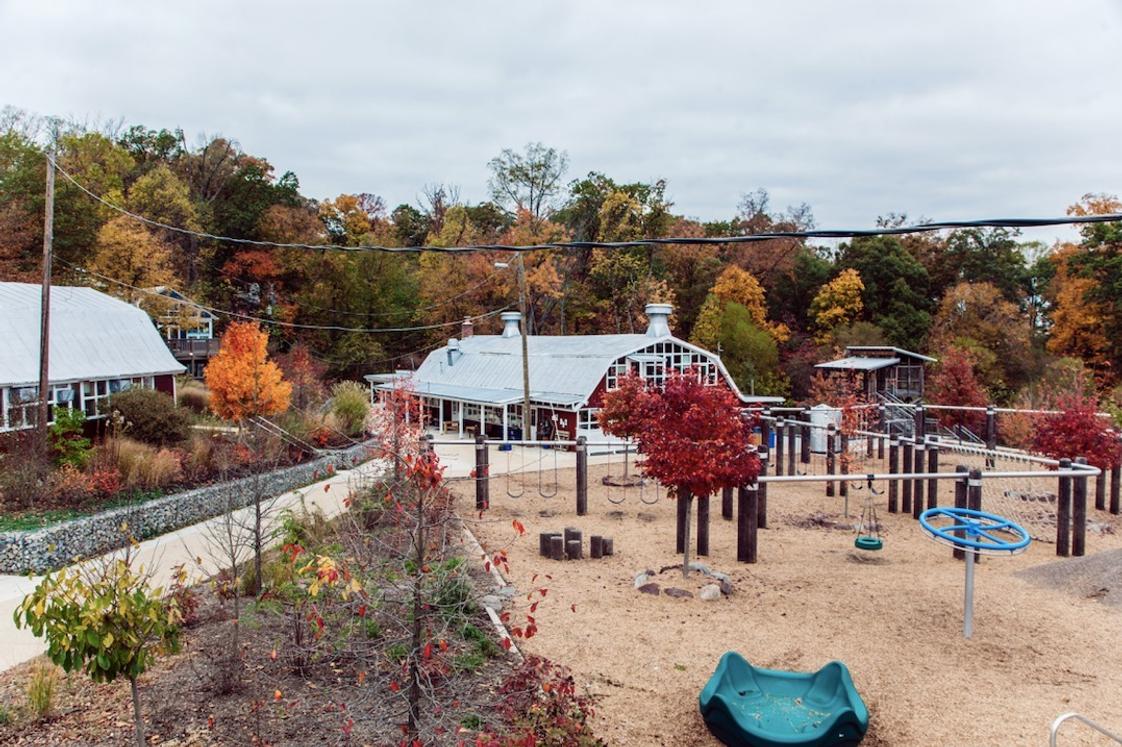The image depicts a vibrant children's playground set against a clear, daylight background. The playground features two sets of swings, a circular blue structure with a pole, and other assorted play equipment, all set on a sandy ground. To the side, there is a striking tree with red leaves, compartmentalized by rocks, evoking a fall season with its mix of green, yellow, orange, and red foliage. In front of the playground, a red house with a gray roof can be seen, accompanied by another similar-colored building to the left. The landscape includes several trees with autumnal colors and a series of electrical poles and wires stretching across the image. The backdrop includes more residential buildings with large glass windows and white roofs, blending seamlessly with the natural surroundings. The sky is a mix of blue and white, adding to the serene atmosphere of the scene.